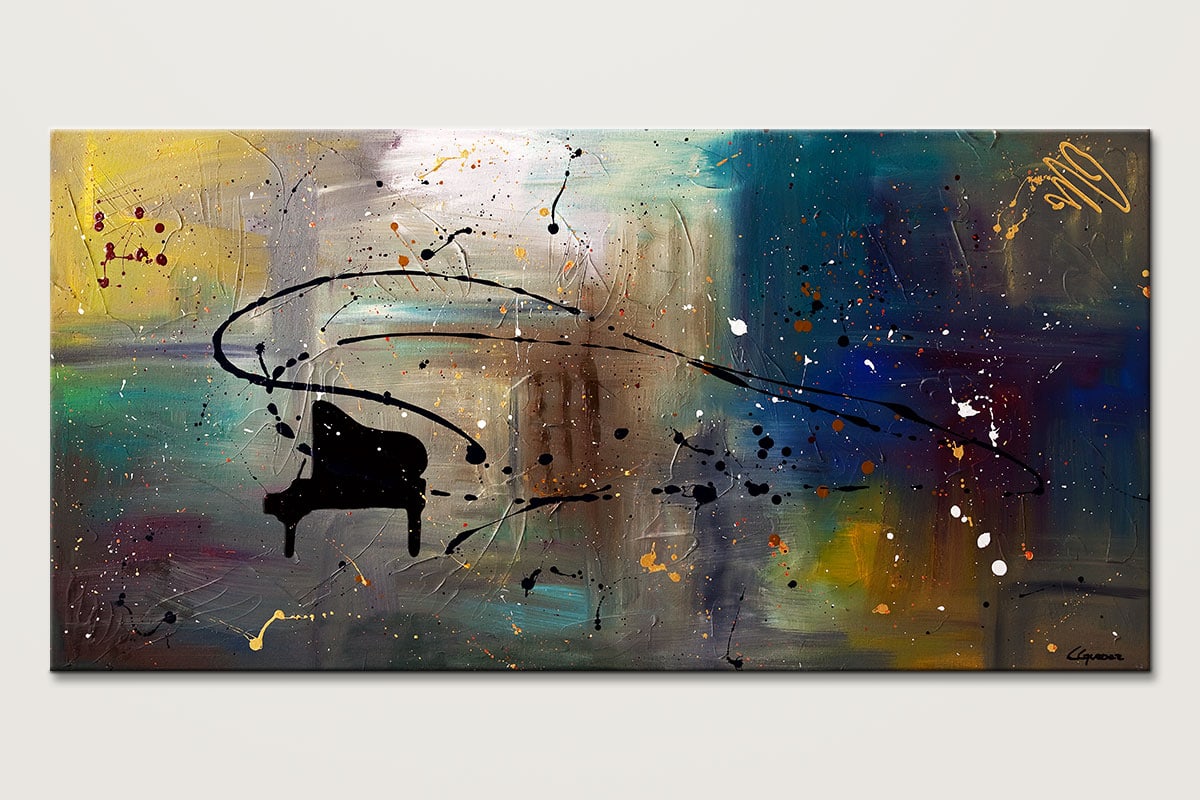This image features a vibrant, multicolored abstract painting displayed on a white wall, capturing a carefully blurred and textural background. Dominating the canvas is a striking black silhouette of a grand piano viewed from the side, clearly showcasing the keys, the open top, and the elegant legs of the instrument. The background consists of thick brushstrokes in an array of colors—yellow, white, green, blue, and hints of red, enhanced by additional splashes of white and gold. There's also a distinctive splatter of paint that seems deliberately dripped across the canvas, adding an extra layer of abstract complexity. The overall composition evokes the impression of blurred fields of color, as if capturing a photograph where the background has been powerfully defocused, highlighting the piano silhouette as the focal point amid the dynamic and colorful backdrop.